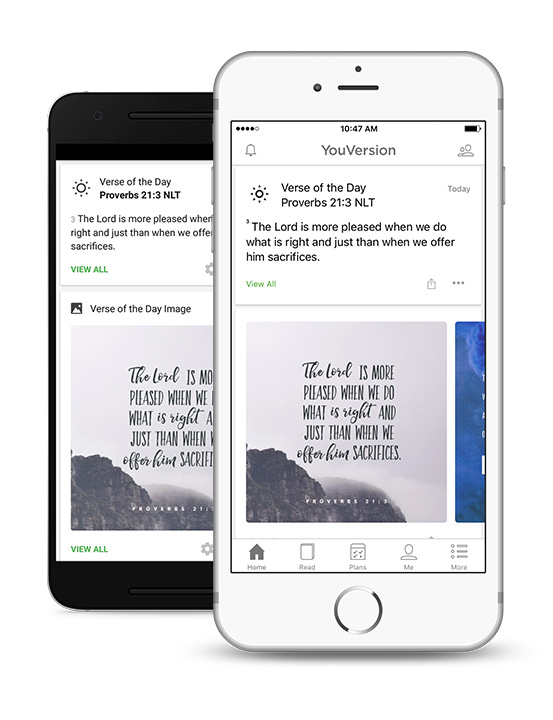The image displays two mobile phones stacked on top of each other. The phone in the background is black and has its screen turned on, showing a social media post. The first post on the screen is titled "Verse of the Day: Proverbs 21:3 (New Testament)" and contains a quote from the Bible. The second post displays a black-and-white landscape photo with an overlaid quote and a "View All" link at the bottom left corner.

The mobile phone on top partially covers the black one and appears to display the same screen. At the top of this phone screen, the line "YouVersion" is visible. The "Verse of the Day" post shows the same Bible verse, Proverbs 21:3 (NLT), with the complete quote: "The Lord is more pleased when we do what is right than when we offer him sacrifices." The landscape photo with the overlaid quote is also displayed, reading: "The Lord is more pleased when we do what is right than when we offer him sacrifices."